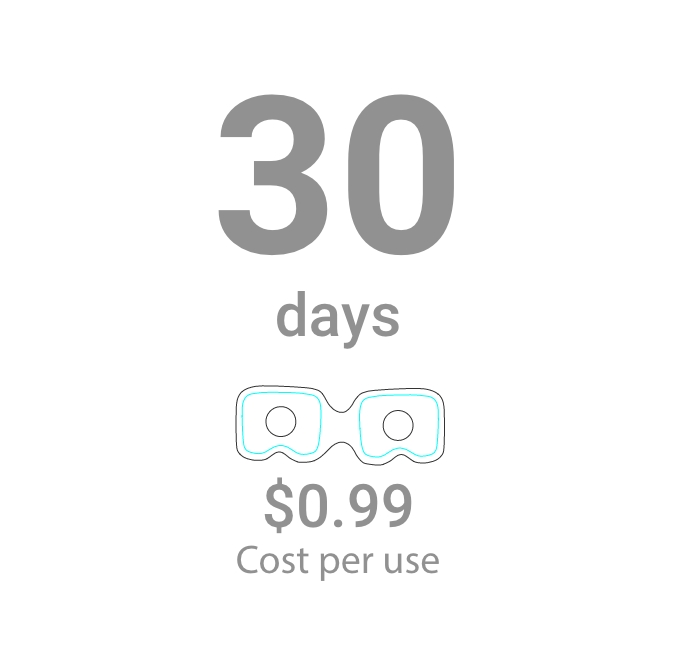The image features a prominently displayed gray number "30," with both digits being approximately three inches in height. Positioned about two inches below this number is the word "days," written in lowercase letters. Below the text are two square shapes with rounded bottom edges resembling a pair of cutout eyeglasses. Inside each of these squares is a blue outline and further within, a black circle, giving the impression of lenses. Beneath this graphic, a price of "$0.99" is shown in black text, followed by the phrase "cost per use." Thus, the entire message conveyed is "30 days, $0.99, cost per use."